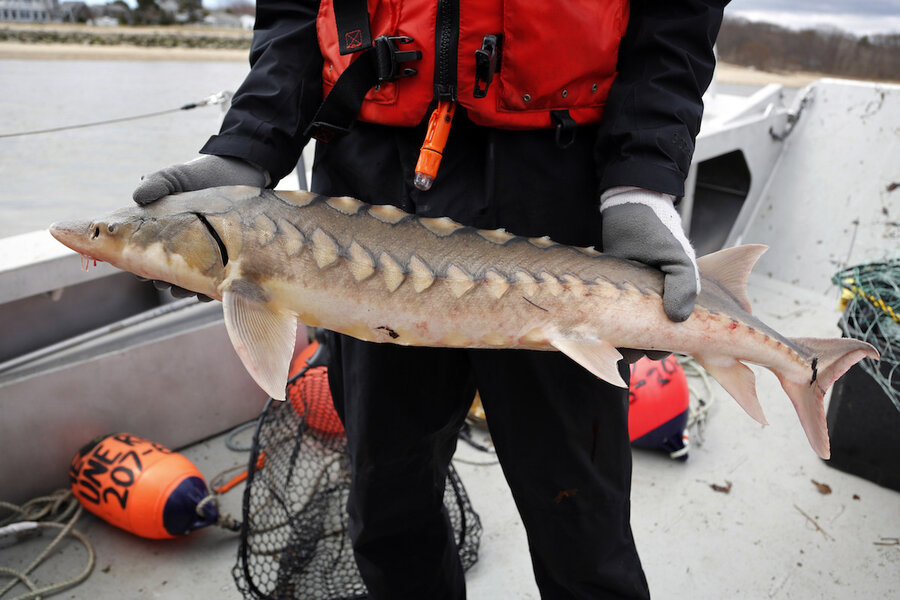In this image, a man clad in black pants, a black long-sleeve coat, protective rubber gloves, and a red safety vest holds a fish on a fishing boat. He was photographed holding what appears to be a baby sturgeon, about three feet long, characterized by large, spiny scales along its sides and top. The fish, with its distinctive spikes, could almost be mistaken for a strange, computer-generated creature due to its unique appearance. In the background, you can see several buoys and fishing nets, indicating that the fish was likely caught in one of the nets. The boat's white bottom is visible, and beyond the vessel, the water stretches towards a shoreline dotted with trees, houses, and other buildings.